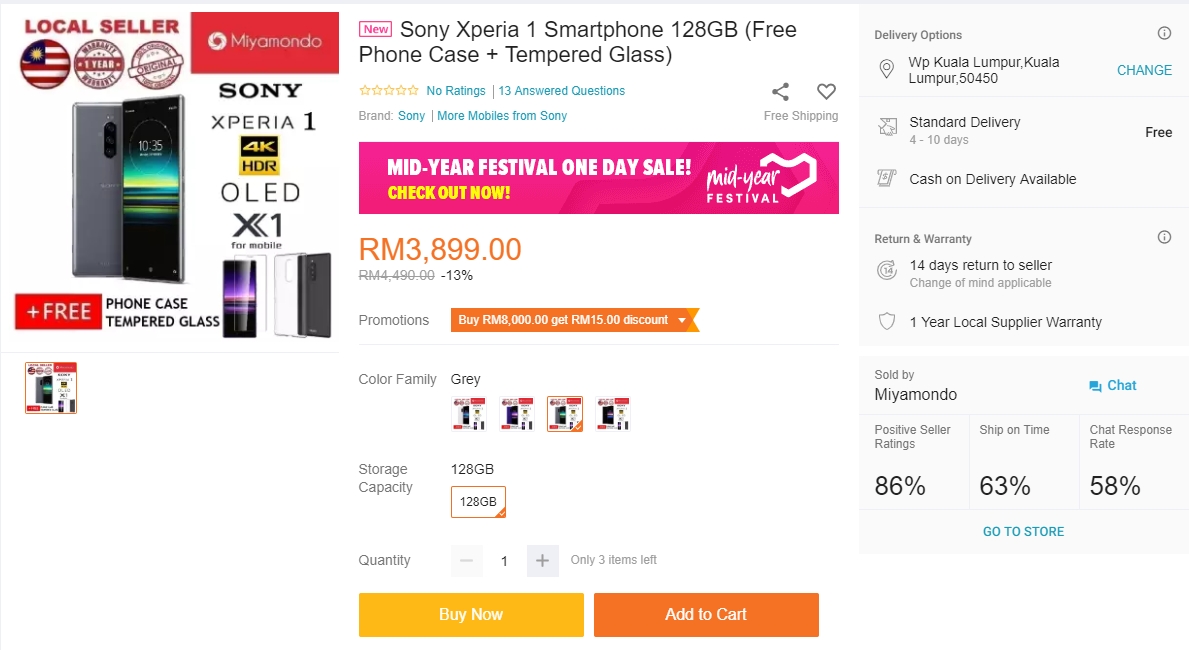This image depicts an online shopping website featuring a detailed listing for a Sony Xperia 1 smartphone against a white background. On the left side, there's a small image of the Sony Xperia 1 phone, adorned with various labels such as "Local Seller," "One-Year Warranty," and mentions of a free phone case and tempered glass included with the purchase.

To the right of the image, a prominent heading announces "New Sony Xperia 1 Smartphone 128 GB" with a note about the included freebies. Directly below this heading are options to view ratings, which currently stand at zero, and 13 answered questions about the product.

Further down, there's a section highlighting the brand "Sony," with an invitation to explore more mobile phones from the same brand. Below this, a small advertisement banner promotes a "Mid-Year Festival One Day Sale," encouraging users to check out the limited-time offers.

The next section displays the phone's cost, prominently showing the sale price of RM 3,899, down from the original price of RM 4,490. A "Promotions" section follows, featuring a small promotional banner. Customers can then choose the phone's color and storage capacity from the available options.

Finally, at the bottom of the listing, two action buttons are present: "Buy Now" and "Add to Cart." 

On the right-hand side of the page, a gray window contains detailed information about the delivery address, estimated delivery time, payment options including cash on delivery, return and warranty policies, seller ratings, and the shipping timeframe.